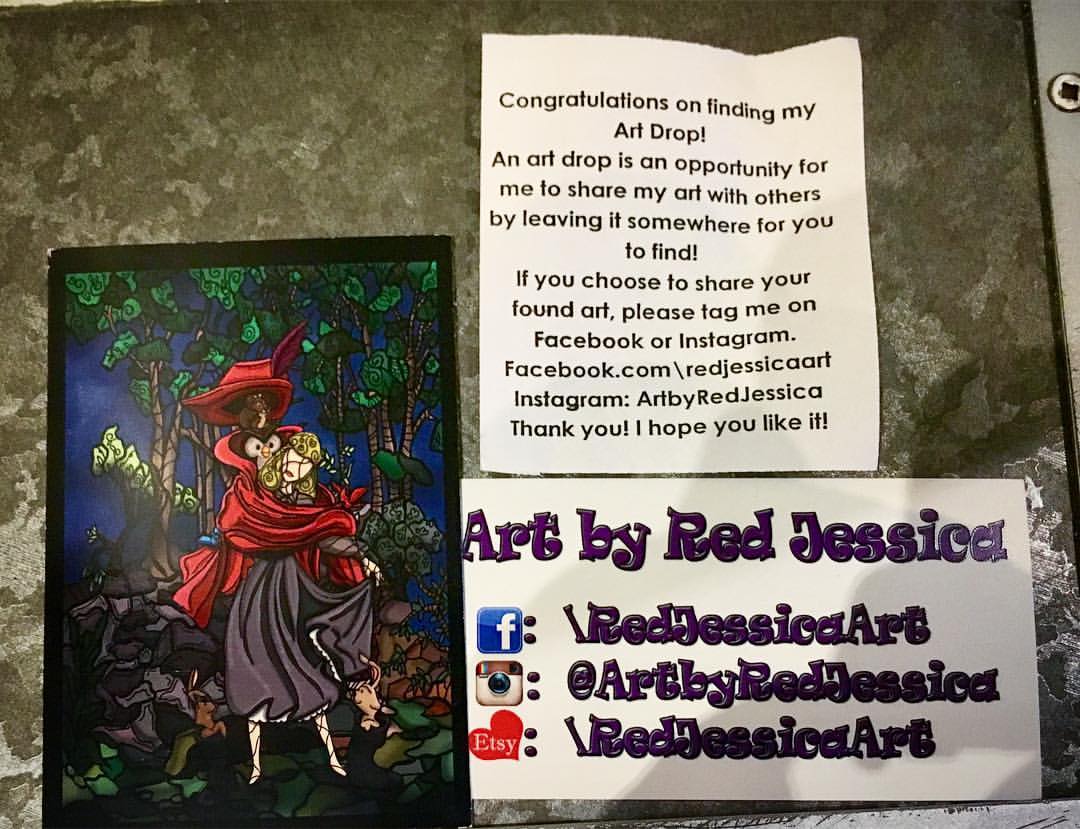This photograph captures a vibrant bulletin board featuring multiple pieces of paper, prominently showcasing an art piece by an artist named Red Jessica. At the core is a small marker painting with a bright, cartoonish, and almost stained-glass quality. The artwork portrays a figure draped in red and gray robes, possibly a princess, adorned with an owl and a rabbit atop her head and shoulders amidst lush, colorful vegetation.

Adjacent to this charming artwork, there are two informative notices. A central piece of paper, slightly above and to the right, enthusiastically announces, "Congratulations on finding my art drop. An art drop is an opportunity for me to share my art with others by leaving it somewhere for you to find. If you choose to share your found art, please tag me on Facebook or Instagram." This message is reiterated with URLs for her social media profiles, encouraging discoverers to share the joy of their find. Below this, another paper reiterates, "Art by Red Jessica," and lists her links to Facebook, Instagram, and Etsy, using a bold, handwritten-style purple font for an inviting touch. The artwork and notes collectively create a whimsical and engaging experience for anyone passing by.